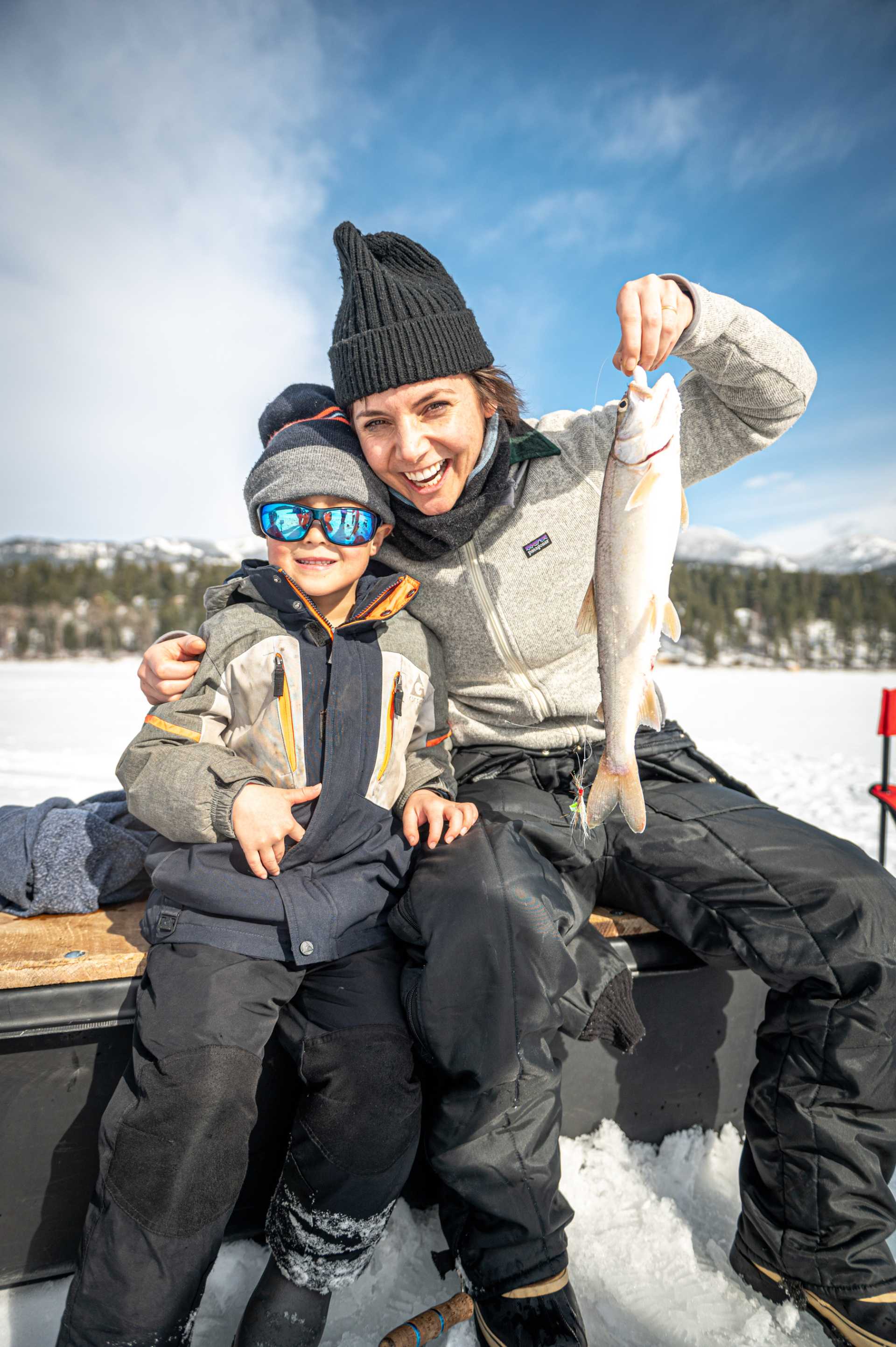In this heartwarming ice fishing scene, a woman and a young boy, possibly mother and son, are seated on a small bench boasting a black base and a light wood-colored top. They are bundled up in winter gear, perfect for the snowy landscape around them. The woman, on the right, wears long black snow pants, black boots, a light gray zip-up sweater, and a black beanie. Her left hand proudly grips a freshly caught fish by the mouth, while her right arm lovingly wraps around the boy. She smiles widely at the camera, her teeth showing. The boy, seated to her left, sports black snow pants, a gray and dark blue coat with colorful trims, blue reflective sunglasses, and a black and gray beanie. He smiles brightly, echoing the woman's joy. Surrounding them is a winter wonderland with snow-covered ground and trees, majestic snow-capped mountains in the distance, and a bright blue sky with a few wispy clouds overhead. The sun casts a cheerful shine over the serene and chilly scene, capturing a perfect, sunny day outdoors.